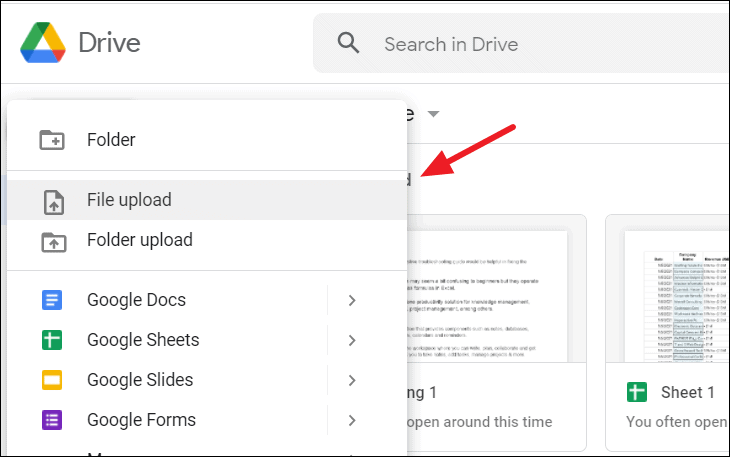The image features a white background with a Google Drive interface prominently displayed. At the top left corner, there's a recognizable Google Drive logo, followed by the word "Drive" written to its immediate right. Adjacent to this, towards the right, is a search bar with a magnifying glass icon and the placeholder text "Search in Drive."

Below this header section, on the left side, there is a vertical column of drop-down menu options. The top menu reads "Folder," followed by consecutive options labeled as "File Upload," "Folder Upload," "Google Docs," "Google Sheets," "Google Slides," and "Google Forms." A red arrow is pointing specifically at the "File Upload" option, indicating it as a point of interest.

In the obscured background of this menu column, there appears to be a partially visible document. On the left side behind the drop-down menus, a sheet of paper is somewhat discernible, though mainly obscured by the aforementioned menus. Certain text elements from this document are visible, including a section where the number 1 and the phrase "Open Around This Time" can be seen. Below this, there is some discernable text that reads "Sheet 1" followed by "You Often Open." Additionally, a block of text with several blue hyperlinks runs down the middle of this largely illegible document. The overall impression is of a busy and somewhat cluttered interface, making detailed elements difficult to distinguish.